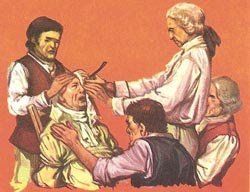This small illustration, set against an orange background, depicts five men during colonial times, characterized by their powdered wigs and period attire. The central focus is on a medical procedure being performed. The most prominent figure is a man on the right, standing and wearing a white shirt and a white powdered wig tied with a ribbon, reminiscent of George Washington or Thomas Jefferson. He appears to be a doctor, holding a gauze pad and an instrument, possibly a knife, as he operates on a bound man’s left eye.

The patient, who is secured to a wooden chair with ropes around his chest and arms, is wearing a yellow shirt. His head is being steadied by another man in a red vest and white shirt with dark hair, positioned on the left-most side. Nearby, a man with dark hair, dressed in a black vest and pink shirt, has his sleeves rolled up, indicating his involvement in the procedure. Another observer with a grey powdered wig, red vest, and white shirt sits in the background, adding to the scene's tension and antiquity. This detailed portrayal vividly captures the somber atmosphere of an 18th-century surgical operation.